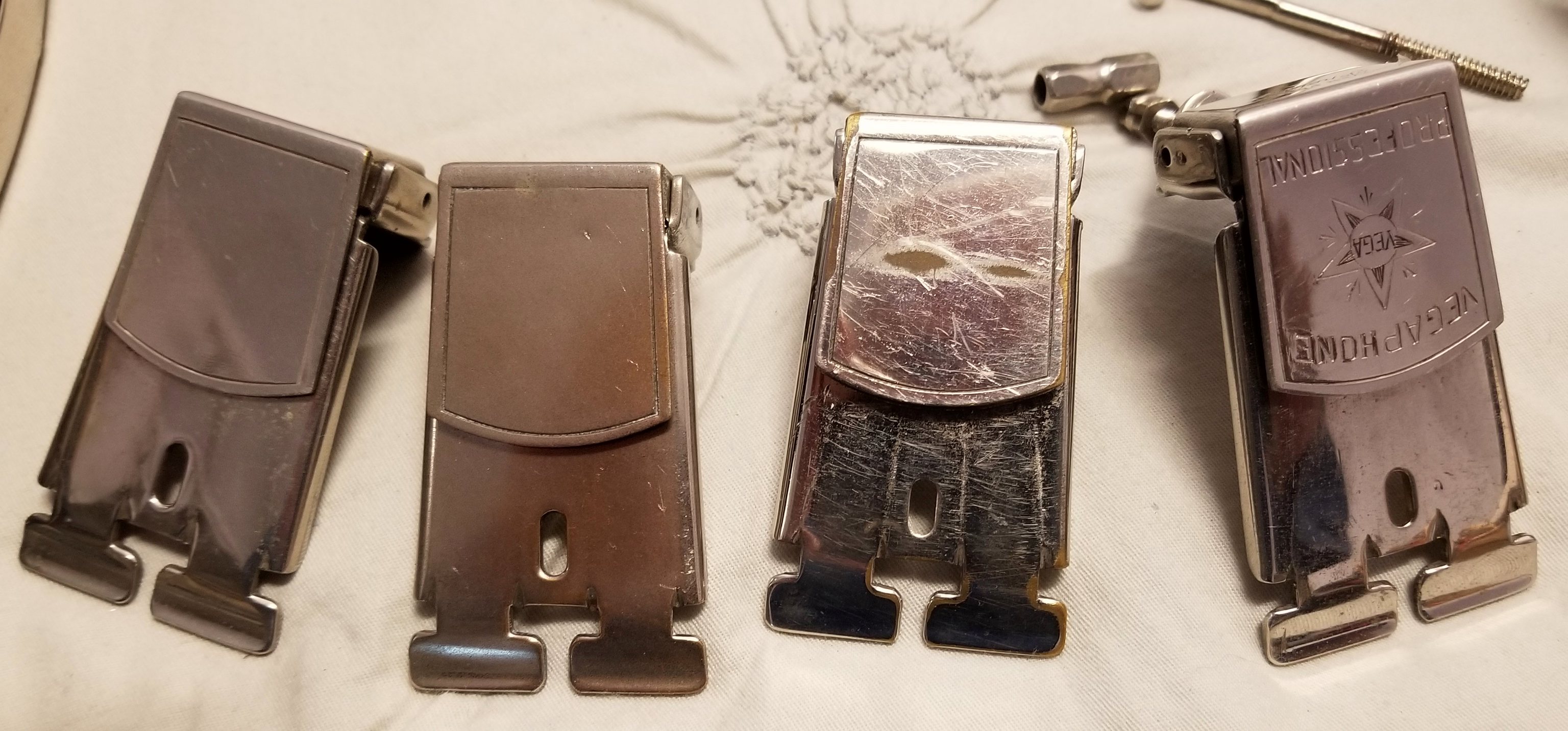The image is a color photograph of four shiny metallic objects, displayed side by side on a white fabric background. These objects, which might be belt buckles or money clips, are made of brass and have a copper-gold sheen enhanced by the camera flash. The fabric features an embroidered light gray flower emblem, centered behind the two middle pieces. Each object has an overlapping flap with a rounded edge on the top half, while the lower half features an oval hole and two protruding stubs with a narrower neck and broader rectangular ends. The item on the far right has an inscription with the word "VEGAS" and a star emblem that reads "Professional" within the center. In the background, some other metallic objects can be seen, including a threaded shaft and couplers.